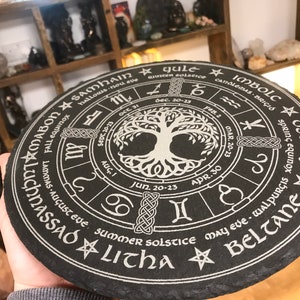The photograph features a person holding a circular disc, possibly made of stone, colored gray with intricate white or light beige graphics. Central to the design is a carved Tree of Life, encircled by the zodiac symbols in a circular pattern denoting the months, further divided by seasonal segments. Surrounding these symbols are inscriptions of various pagan holidays such as "Summer Solstice," "Litha," "Beltane," "Yule," and "Samhain." Additional Celtic cross motifs are also present along the perimeter. The disc is being held by someone wearing a sweater, with only their hand visible. The background reveals shelves filled with knickknacks, including what appears to be crystals or stones, and a brown table beneath the object.